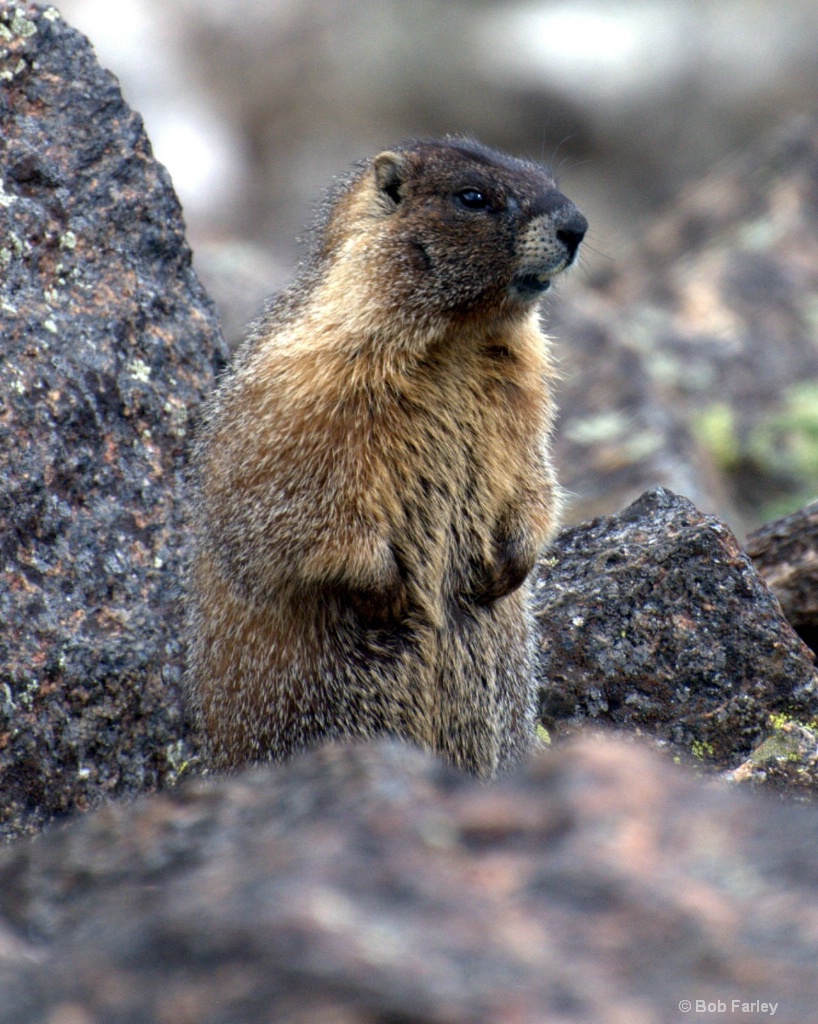In this image, we see a small furry creature, possibly a groundhog, standing on its hind legs in the center of the frame. The animal has light to medium brown fur with a darker brown area around its face. Its tiny front paws are visible, held slightly in front of its body, and its small ears are also noticeable. The creature is oriented towards the 3 to 4 o'clock position, seemingly focused in that direction.

The background and foreground are both blurred, highlighting the main subject but suggesting a rocky environment. The surface the animal stands on is composed of dark brown rocks, speckled with orange and white, resembling a miniature mountain range. These rough, peaking rocks extend behind and around the creature, giving the impression of a rugged outdoor setting.

The color palette of the image includes various shades of brown, black, white, orange, gray, and green. Notably, the photograph features a copyright label that reads "Bob Farley." The overall composition suggests the image was captured outdoors, possibly by a hidden camera.